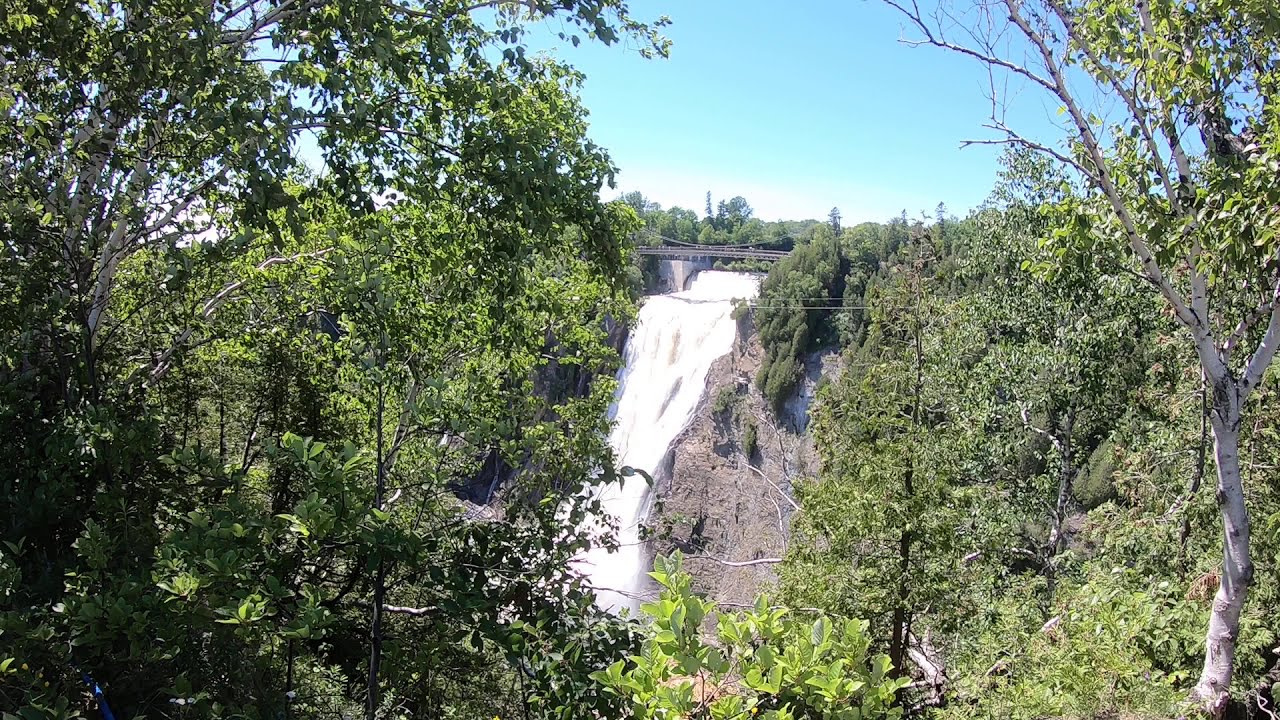In this breathtaking nature scene, a majestic waterfall cascades down the center of a rugged brown cliff, framed by lush green foliage and trees on both sides. The top of the image features a serene light blue sky, gradually transitioning to white near the horizon. Prominently, a rustic brown wooden bridge with suspension ropes spans the cliff just before the waterfall begins its descent. Surrounding the scene are various thin, white or dark brown-trunked trees laden with green leaves, partially obscuring the view. Large rocks at the base add to the wilderness atmosphere. A wire crosses the image just above the lower portion of the waterfall, adding a subtle human element to the predominantly natural environment. The distant perspective emphasizes the vastness and tranquility of this picturesque landscape, capturing the essence of unspoiled nature.